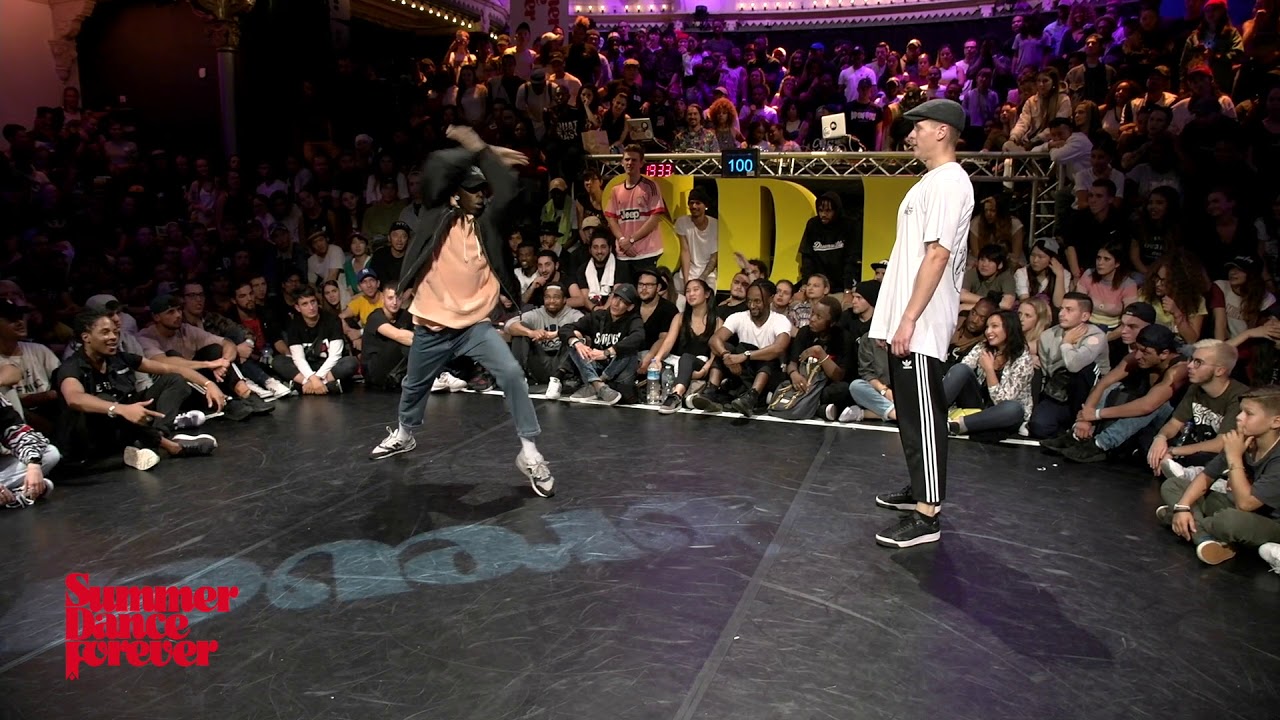A captivating photograph from the "Summer Dance Forever" event, as indicated by the red watermark in the bottom left corner, captures a vibrant dance battle. Center stage, a relatively small black platform, is flanked by a wide array of diverse audience members seated on the floor. In the foreground, a Black man, dressed in a black baseball cap, yellow sweater under a black jacket, slacks, and New Balance sneakers, is mid-movement, executing a dynamic dance pose with arms raised and legs positioned for balance. To his left, a white man in Adidas sweatpants, black shoes, an oversized white graphic tee, and a beret, watches intently, possibly awaiting his turn. Elevated in the background is another group of audience members, some seated and some standing, who occupy a podium area. Prominently displayed on this raised section are large yellow letters suggesting the presence of judges alongside two electronic clocks, one displaying "100" in blue and the other "1933" in red. The image pulsates with energy and excitement, embodying the spirit of a live dance-off in a packed venue.